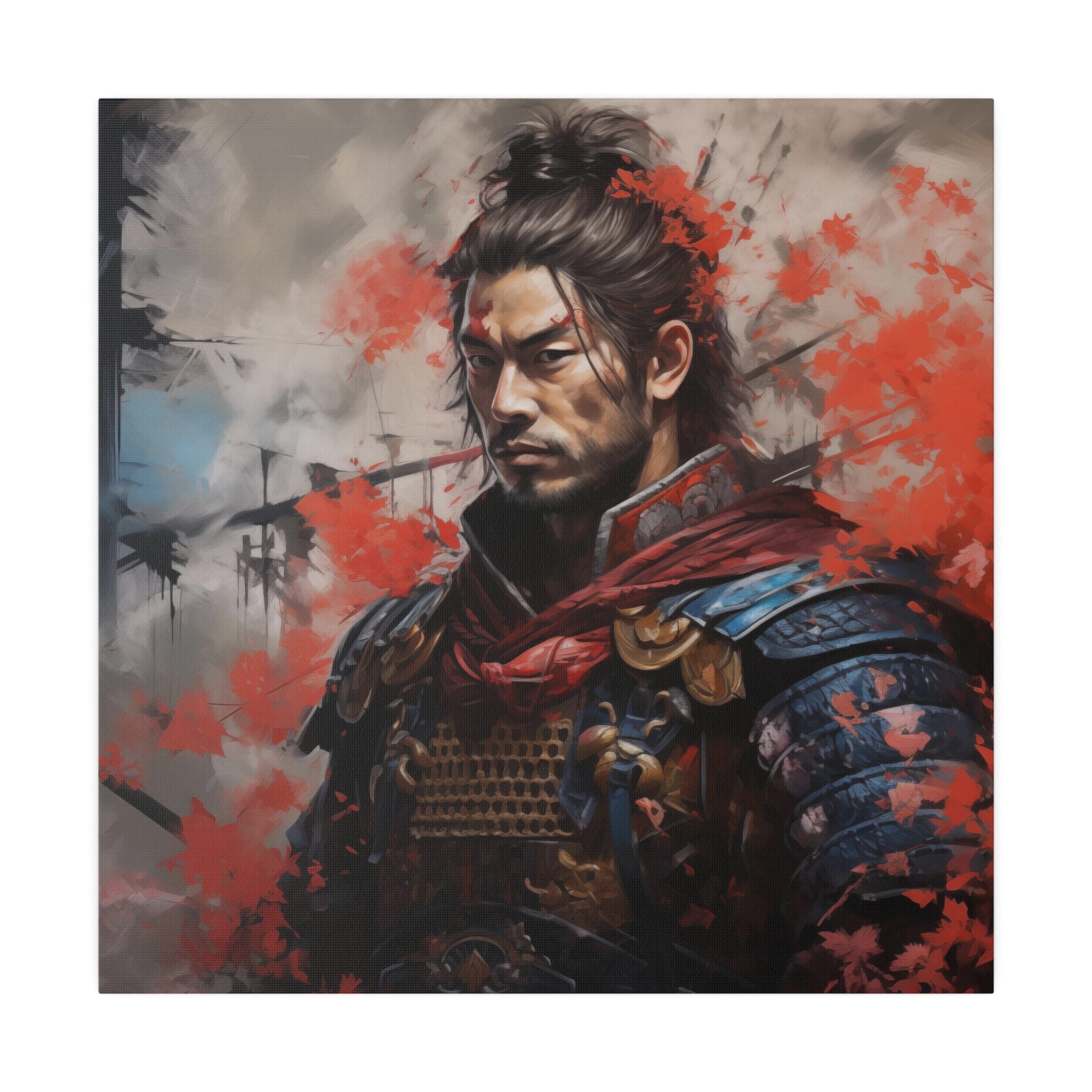This hyper-realistic painting portrays an ancient samurai warrior standing at a slight angle, with his right shoulder turned back and left shoulder forward. His stern face, accentuated by scowling eyebrows, a thin mustache, and a goatee, reflects a fierce determination. Long black hair is pulled up into a bun, with stray strands adding to his rugged appearance. Blood splatters mar his face, hair, and the surrounding gray, smoky background, intensifying the chaotic scene. Dressed in ornate armor, the samurai wears a blue suit with a red collar and silver accents. His chest piece features gold half-circle attachments connecting the shoulder pads and a hexagonal wicker pattern adorned with matching straps. A prominent red cape ties at the front, adding grandeur to his formidable presence. Behind him, a flurry of arrows and spikes punctuates the air, enhancing the battlefield atmosphere. The left side of the background tinges blue, while the right side is speckled with red, further highlighting the tumultuous setting.